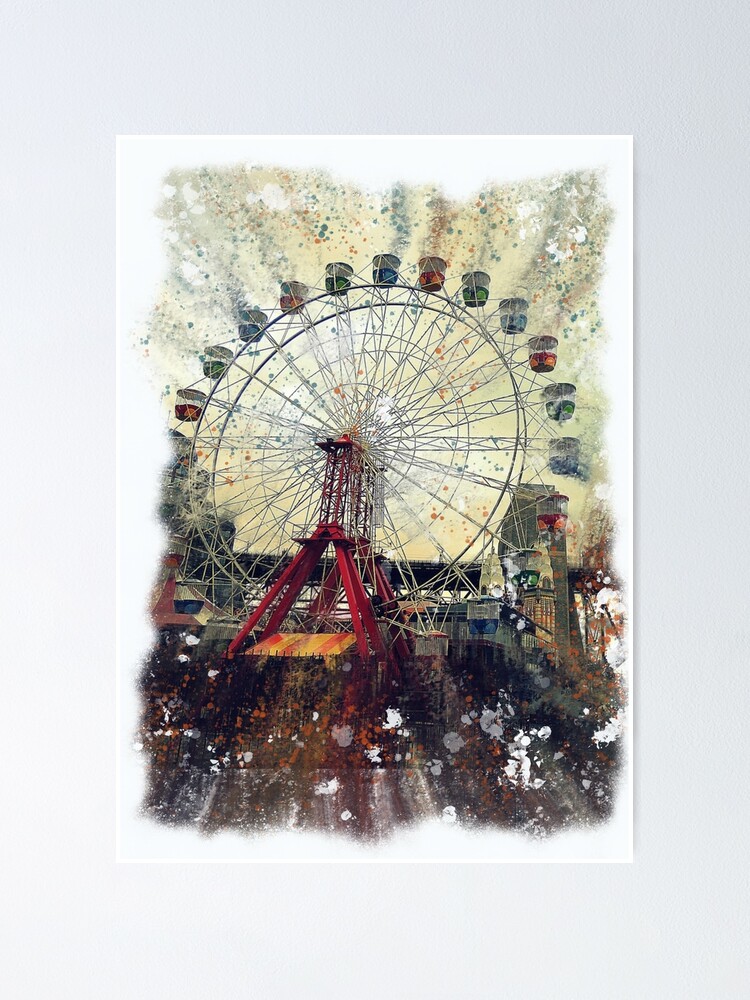This image is a detailed, color illustration of a large, vintage-style Ferris wheel, likely created with watercolor techniques. The Ferris wheel stands prominently on its own, drawing attention due to a slightly blurred and speckled cream-colored background with dots that distort the surroundings, emphasizing the wheel itself. The base of the Ferris wheel is a vibrant red A-frame, transitioning into a red and orange platform below. The wheel's structure includes silver spokes supporting gondola-style seats of varying colors, including red, green, gray, and blue, covered canopies running along the top. The artwork blends browns at the bottom and grays at the top, with hints of trees suggesting an urban setting, although details remain abstract and indistinct. The illustration's border is unfinished, and no text is present.